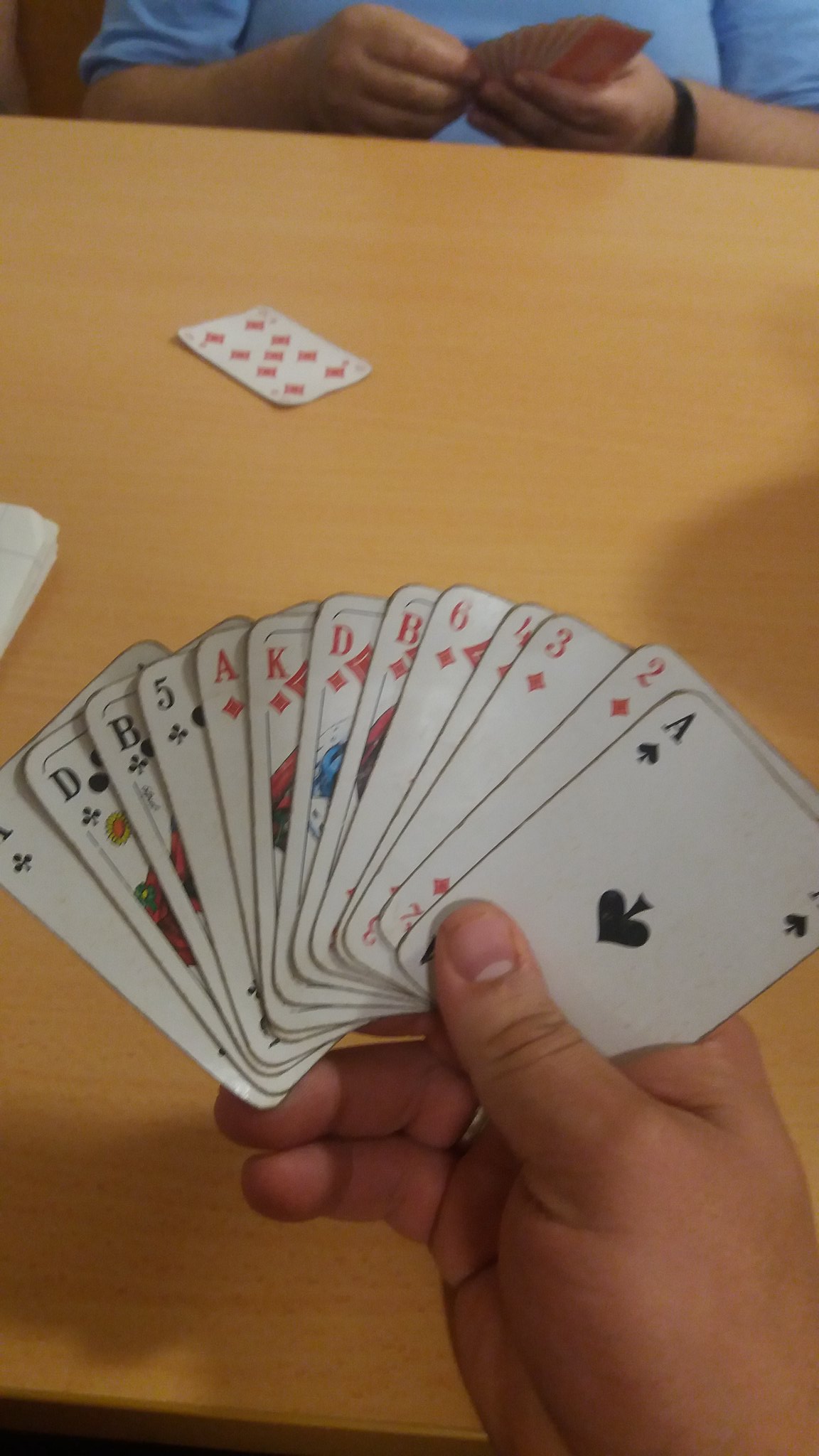This indoor color photograph captures a light brown wooden table with prominent wood grain. On one side of the table, the hands and forearms of a man are visible. He is wearing a blue t-shirt and a black wristwatch. The man's left hand holds a fan of seven or eight playing cards with red backs. A single card, identified as the nine of diamonds, lies face-up on the table in front of him.

Opposite the man, only a single right hand is visible, holding a spread of playing cards. This hand displays cards with an odd assortment that includes an ace, a two, a three, a ten, a six, and various other cards, including some with letters 'B' and 'D'—anomalies suggesting the possibility of an AI-generated image, as traditional playing cards do not feature such characters.